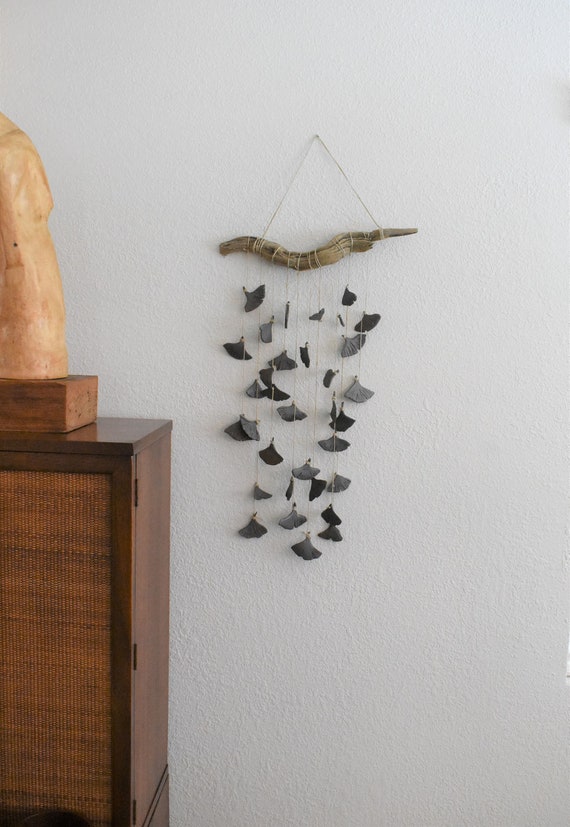The photograph depicts a unique piece of wall art hanging against a white plaster wall. At the top, a twisted or curved piece of driftwood serves as the anchor, from which various strands of twine descend. The twine is meticulously arranged to form a loop, securing the art to a nail on the wall. Hanging from the twine are multiple pieces designed to resemble a mobile; these pieces are light and dark gray, vaguely diamond-shaped and reminiscent of inverted fan shapes, possibly made of clay. The arrangement gives the piece a delicate, wind chime-like appearance.

To the side, there is a brown dresser. On top of this dresser sits an old-school record player with a stone placed on it. The stone is notably orange and adds a contrasting pop of color to the scene. Additionally, atop the dresser there's a tan-colored sculpture on a wooden base, although it is partially cut off by the edge of the photograph’s frame, adding a sense of intrigue to the composition.